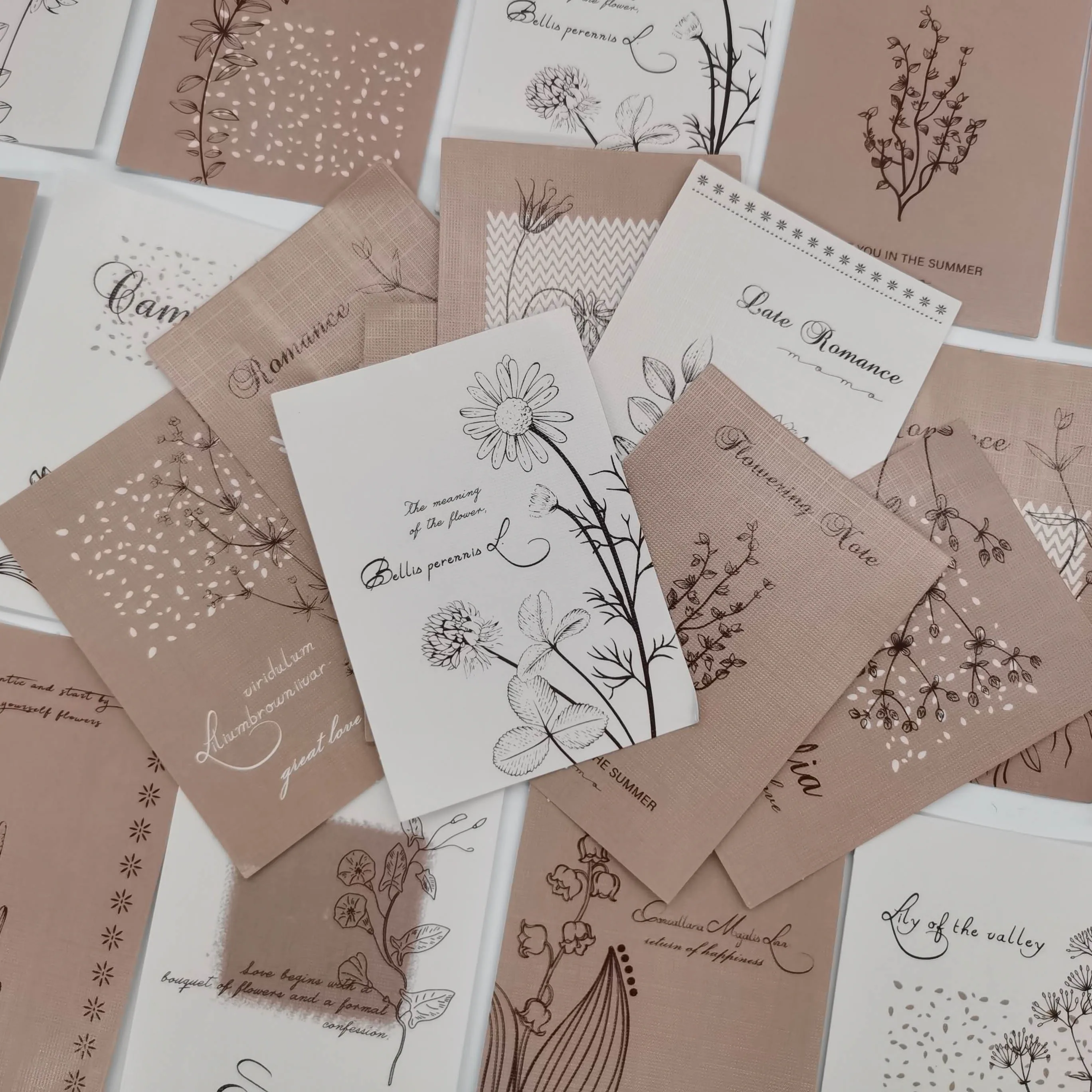This image displays a meticulously arranged assortment of greeting cards, artfully placed on a white table. The cards, adorned with elegant calligraphy in black ink, showcase a harmonious palette of brown, white, and tan hues. Each card features botanical illustrations and romantic messages, often including Latin names of flowers. 

In the center of the image, a white card sits atop the arrangement, prominently displaying a drawing of a daisy flower and leaves. It reads "The Meaning of the Flower" with a Latin name beneath it. Surrounding this central card, a spread of taupe and ivory cards extends in a feathered stack. To the left of the centerpiece, one card on taupe paper reads "Viridulum Lombraun Ivar, Great Love," accompanied by an illustration of a viney plant. To the right, another taupe card situated beneath the front card mentions "Flowering Note" and shows off summer-themed vines and leaves. 

In the bottom right corner, an ivory-colored card details "Lily of the Valley," while another card in the top right corner states, "See you in the Summer." The captions on these greeting cards collectively explore themes of romance, love, and botanical beauty, making for an enchanting, harmonious display.